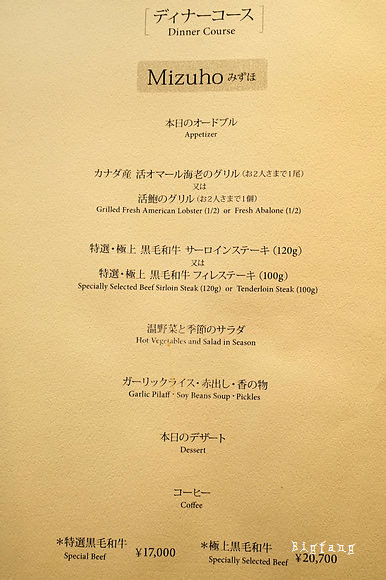The image is a rectangular photograph of a dinner menu, with its left and right sides longer than the top and bottom. In the very bottom right corner of the photo, there is white text that reads "Big Fang." The menu itself is printed on thick cardstock that is a yellowish-tan color, giving it a textured, pit-marked appearance. The content of the menu is predominantly in Japanese, with English translations provided underneath. 

At the top of the menu, in large text, it reads "Dinner Course." Beneath this heading, there is a light gray rectangle containing the black text "Mizuho." The menu lists the following items:

- Appetizer: Grilled Fresh American Lobster Half or Fresh Abalone Half
- Specially Selected Beef: Sirloin Steak 120g or Tenderloin Steak 100g
- Hot Vegetables and Salad in Season
- Garlic Pilaf
- Soybean Soup
- Pickles
- Dessert
- Coffee

The prices for the beef options are also listed: Special Beef for 17,000 Yen and Specially Selected Beef for 20,700 Yen.